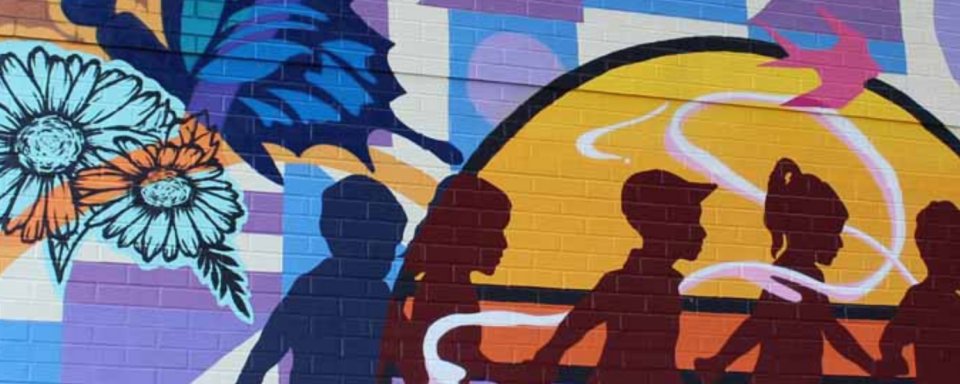The mural, painted on the side of a brick building, showcases a dynamic and colorful scene. In the foreground, the silhouettes of five children, estimated to be around six or seven years old, are holding hands and walking to the right. Their playful movement suggests participation in a children's game. Behind them, a large yellow circular object, possibly representing the Sun, forms the backdrop. The top half of this circle is painted orange, while the lower half transitions to a reddish hue.

Blue and purple geometric shapes dominate the background, overlapping and blending with one another to create a modern and abstract feel. Among these shapes, a pink bird, resembling a dove, flies above the Sun near the upper right corner of the mural, and a blue butterfly perches lightly behind some brightly painted blue flowers on the left side. These flowers are distinctively marked with orange stripes. The entire mural is a narrow rectangular landscape, filled with vibrant colors and a sense of joy and movement, hinting at its role as part of a larger urban art installation. Despite the partial view, the cracks and gaps in the bricks visible behind the artwork affirm its placement on an exterior wall, enhancing the piece's urban charm.